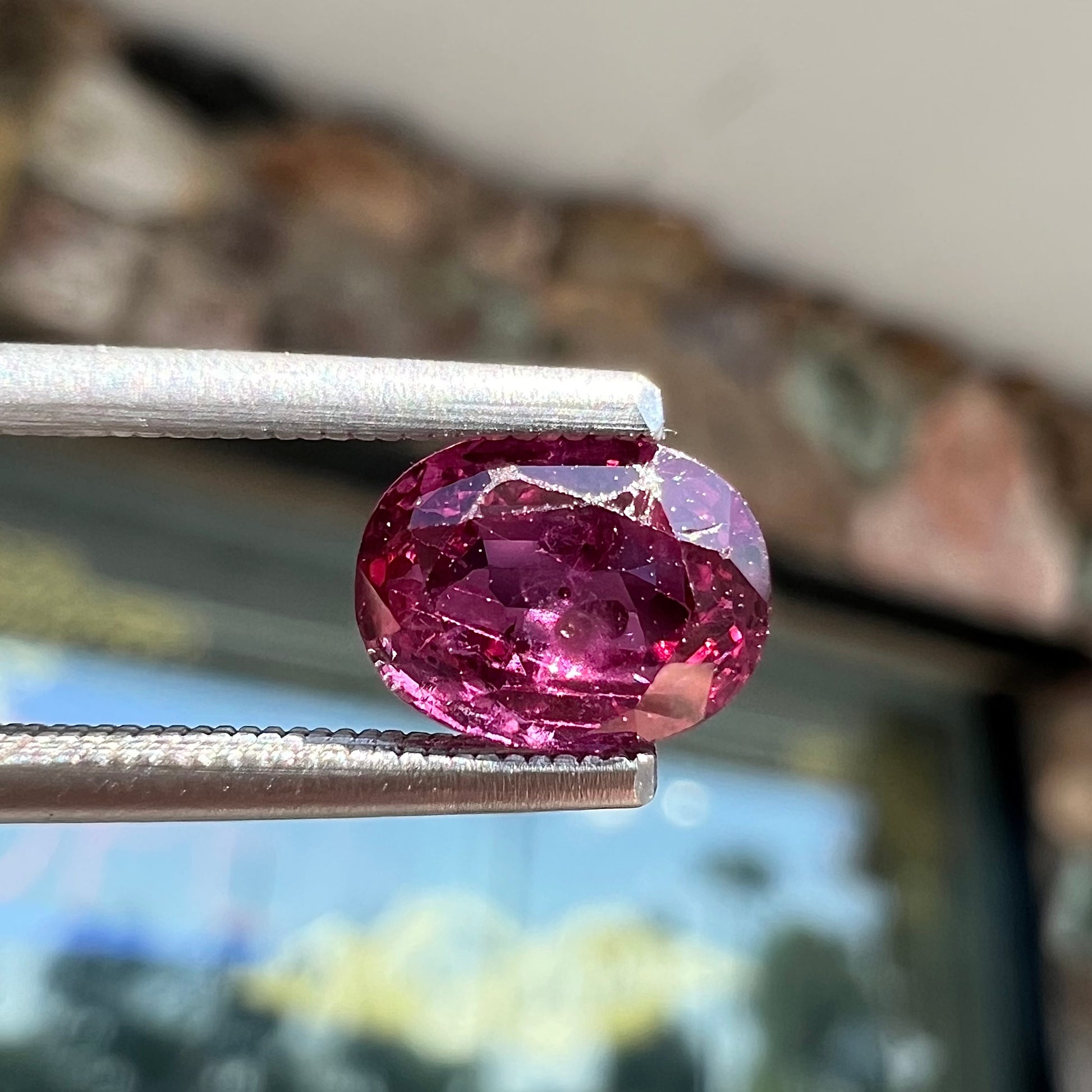In the image, a meticulously cut and polished amethyst, showcasing its characteristic deep purple hue, is held delicately between steel tweezers. The amethyst, shaped into an elegant oval, is prominently positioned at the center of the frame. The tweezers, grasping the top and bottom sections of the gem, extend from the gem to the left edge of the image, gradually fading out of view. The backdrop appears to be an exterior view of a shop, identifiable by a large, somewhat reflective, glass window occupying the bottom left to the center right of the image. Above the window, a stone-topped wall is visible, complete with what looks like pull-down shutters. The background is significantly blurred, suggesting a shallow depth of field, and the presence of daylight is evident from the reflections on both the glass window and the amethyst itself. The sunlight highlights the facets of the gem, adding an extra sparkle to this exquisite piece.